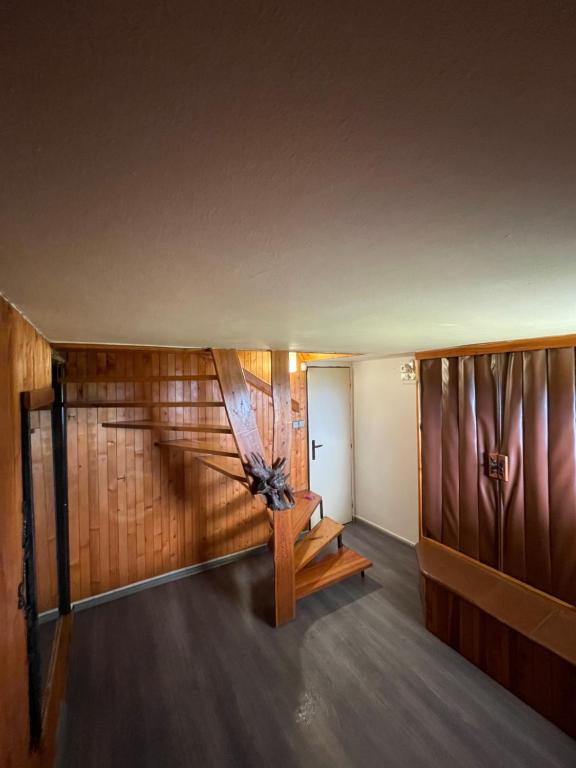This image captures a dimly lit basement room with minimal natural lighting. The room features a low, plastered ceiling and dark gray wooden floors. Central to the image is a curved wooden staircase leading to the upper floor. The walls are predominantly wood paneled in a medium tone, enhancing the basement's cozy yet somewhat confined atmosphere. 

On the left side of the room, a large black-framed mirror is mounted on the wooden wall, and nearby is a door that opens to another room. Adjacent to this door is an off-white section of the wall. Behind the staircase, the wooden walls are segmented, adding a textured look to the background. 

On the right side, there's a curtain or pull-away door, possibly made of dark brown vinyl or leather, that likely conceals a storage area. This section is complemented by surrounding wooden trim. High above a white wall in the background, near the storage space, an emergency light glows, further illuminating the doorway. Additionally, a dark, indistinguishable statue rests on the staircase, adding a touch of intrigue to the scene.